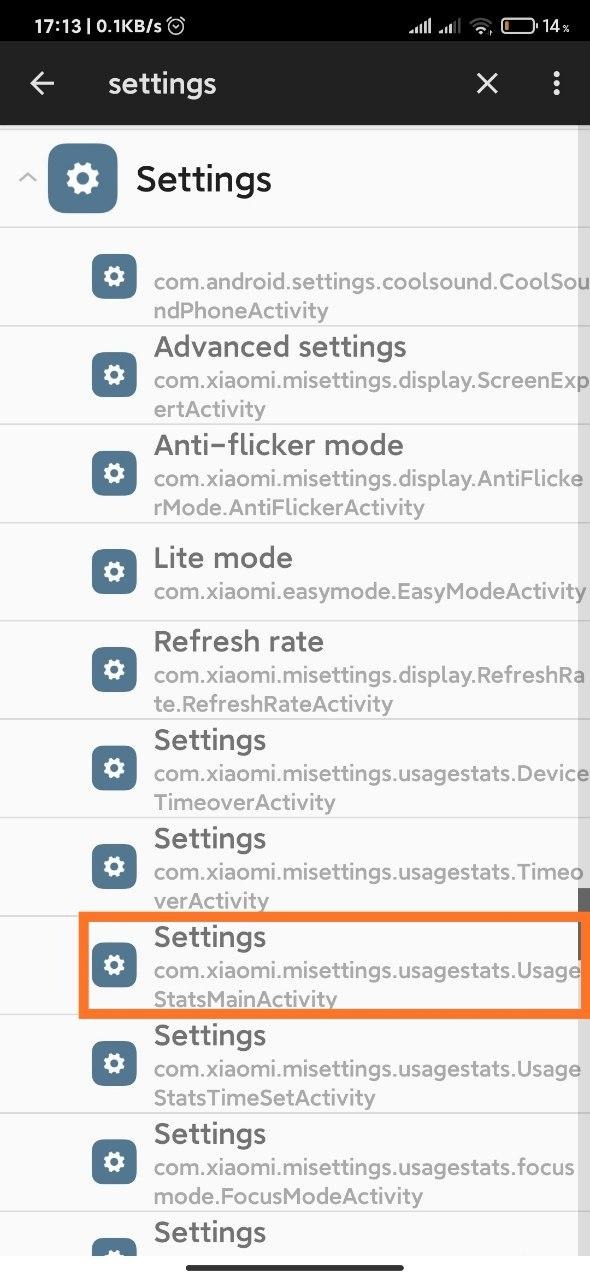This screenshot captures the settings menu of a smartphone. The background is predominantly white, while the top status bar is black, displaying the time as 17:13. The phone exhibits critical details such as 0.1 gigabytes of available storage, a nearly depleted battery at 14%, a very weak Wi-Fi signal, and the volume set to its maximum level. 

In the settings menu, approximately three-fourths down the screen, there is an orange highlight around several options, indicating their selection. These options are boxed separately, with the highlighted selection labeled as "com.vioxami.settings". Interestingly, the last six settings in the menu appear nearly identical, featuring the same descriptive text, making them indistinguishable from one another. Additionally, the clickable icons for these settings are depicted in a very light navy blue.